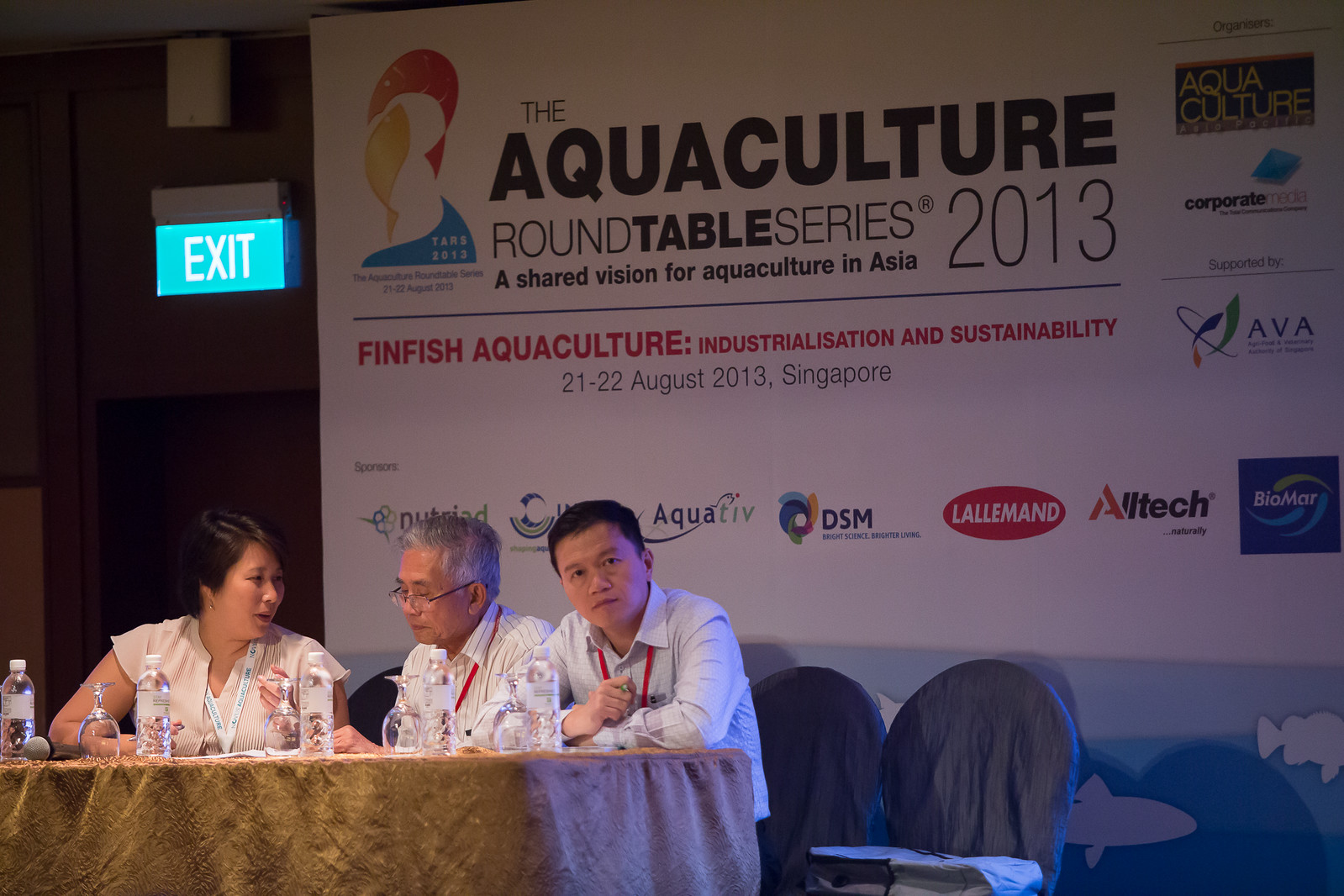This image captures a moment from the "Aquaculture Roundtable Series 2013: A Shared Vision for Aquaculture in Asia," an event focused on FinFish Aquaculture Industrialization and Sustainability, hosted in Singapore from August 21-22, 2013. At the center of the image, three conference delegates are seated behind a light brown cloth-covered table, situated on a podium stage facing what can be presumed to be an audience. On the table are five water bottles and several upside-down clear drinking glasses. Two of the delegates, one a woman and the other an elderly man with glasses and a light-colored floral print shirt, are actively engaged in conversation. The third delegate, a younger man with short hair, appears disengaged and gazes off towards the camera. Each delegate wears a lanyard and a white shirt, with two in long sleeves and one in short sleeves. In the background, a large billboard prominently displays the event's title and dates, along with the names of sponsoring companies. To the left of the billboard, a glowing green exit sign is visible above a door. The room appears dimly lit, suggesting a moment either towards the end of the day's discussions or during a pause in the proceedings.